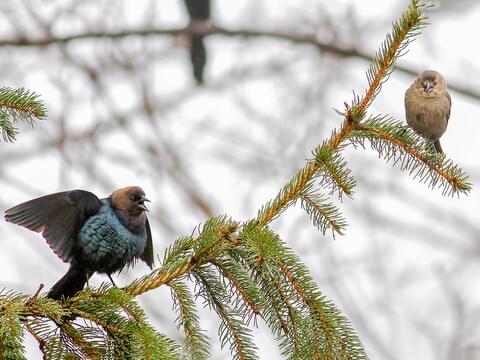The photograph captures a dynamic winter scene featuring two warbler-like birds perched on a branch of a Douglas fir tree. The branch, adorned with green pine needles, stretches horizontally, creating a natural stage for their interaction. On the left side, a male warbler with striking bright blue chest plumage, and black wings extends his wings and puffs out his feathers, his beak wide open as he appears to be chirping or squawking, possibly in an attempt to assert his dominance or defend his territory. In stark contrast, the right side of the branch hosts a more subdued, brown female warbler. Her wings are tucked in close to her body and her beak remains closed, indicating a calm, yet resolute stance. The background features an out-of-focus white sky, suggestive of a wintry atmosphere, though the primary focus remains on the vivid and detailed interaction between the two birds.